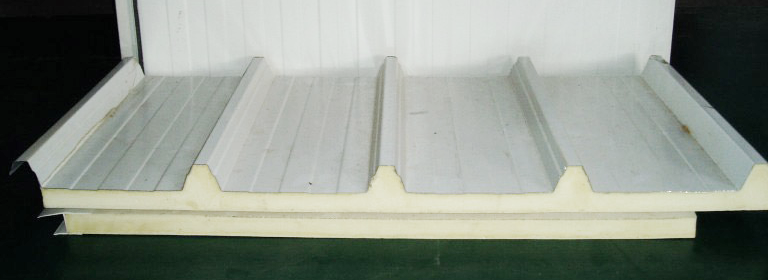The photograph features a rectangular object set against a dark background. The object, primarily white, appears to be an ornately decorated surface divided into four equal lanes, each accentuated by grooves or ridges. These sections likely provide structural support. The item, potentially a piece of furniture or an appliance door—possibly from a refrigerator due to its metallic appearance—is quite old. The image lacks any contextual background or additional objects to clarify its setting. The intricate design suggests it could be used for aesthetic or functional purposes, such as shelving without bookends or insulated roofing material, with a layer that could potentially be foam for insulation. While its exact identity remains ambiguous, the detailed segmentation and the stark contrast between the white object and the dark background make it a striking subject.